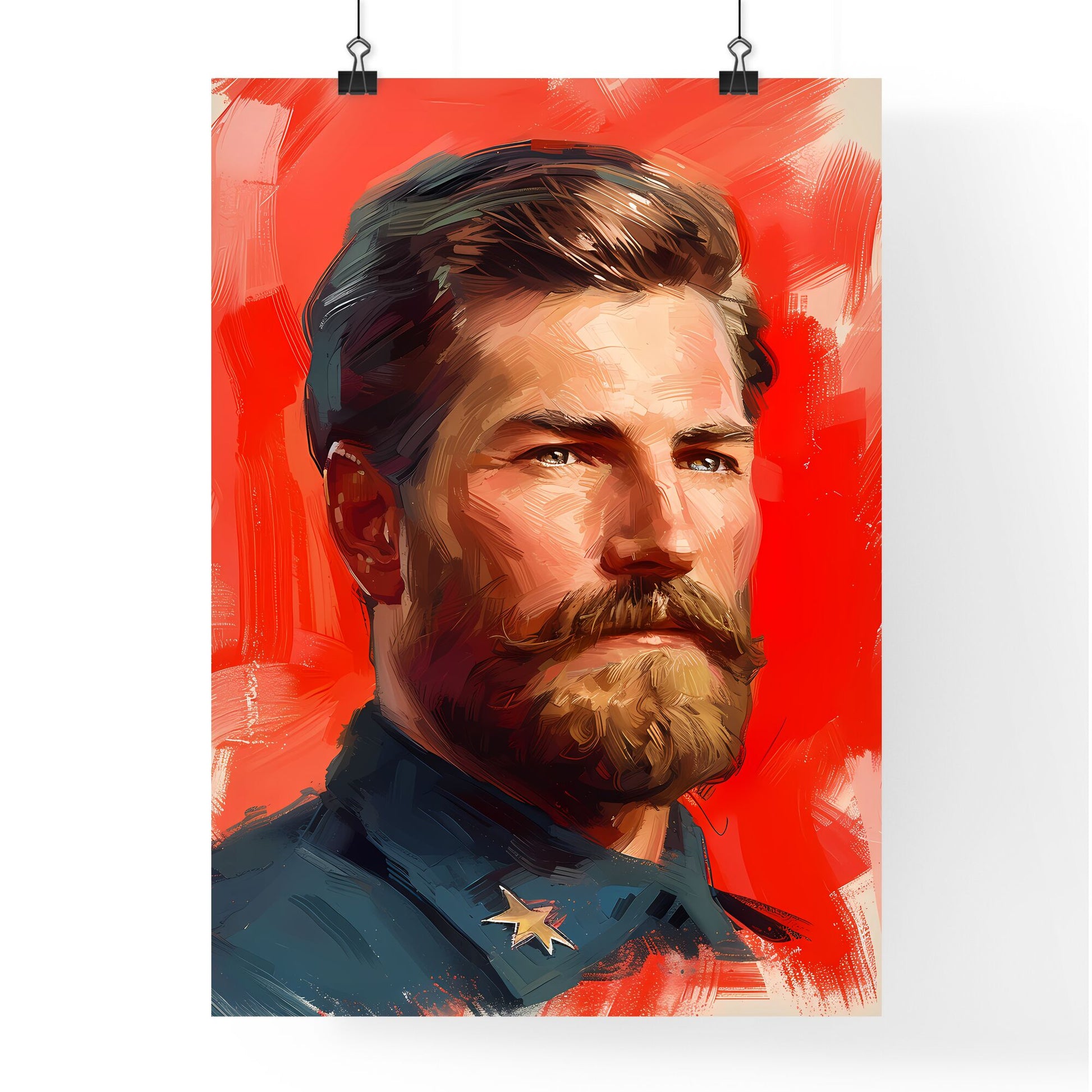This detailed photographic art piece, displayed indoors on a white wall, is suspended by two black clips with silver hooks. The painting features a white man in his 30s or 40s with brown hair parted to the right, sporting a prominent nose, brown mustache, and beard. His eyes are brown, and he gazes slightly to the right, giving a terse expression. The man's ear appears slightly red, possibly hinting at the light source from the right. He is dressed in a blue military shirt adorned with a six-pointed gold star on the left collar. The striking red background is marked with expressive brushstrokes, and there is no text in the image. This head-and-shoulders portrait is a compelling and detailed representation of the subject.